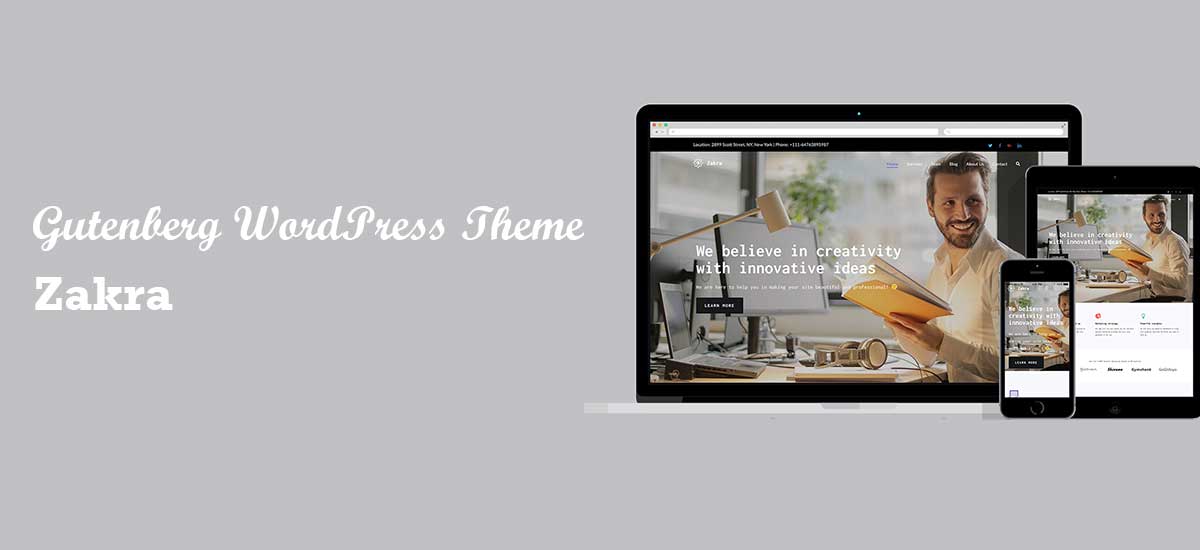The image features a grey background with text positioned on the left. In white cursive font, it reads "Gutenberg WordPress theme," and beneath it, in a different white font, it says "Zakra." On the right side of the image, there are three mockups: a laptop, a tablet, and a mobile phone. The laptop monitor is positioned at the back, with the tablet in front of it, and to the left of the tablet, the mobile phone is displayed.

Each device screen showcases an identical image of a man sitting at a computer, holding a yellow book and smiling. He is wearing a white t-shirt, and the photograph includes overlaid white text that states, "We believe in creativity with innovative ideas." On the tablet screen, there is an additional text box located beneath the main photograph, while the mobile version also shows a partial text box underneath the image.